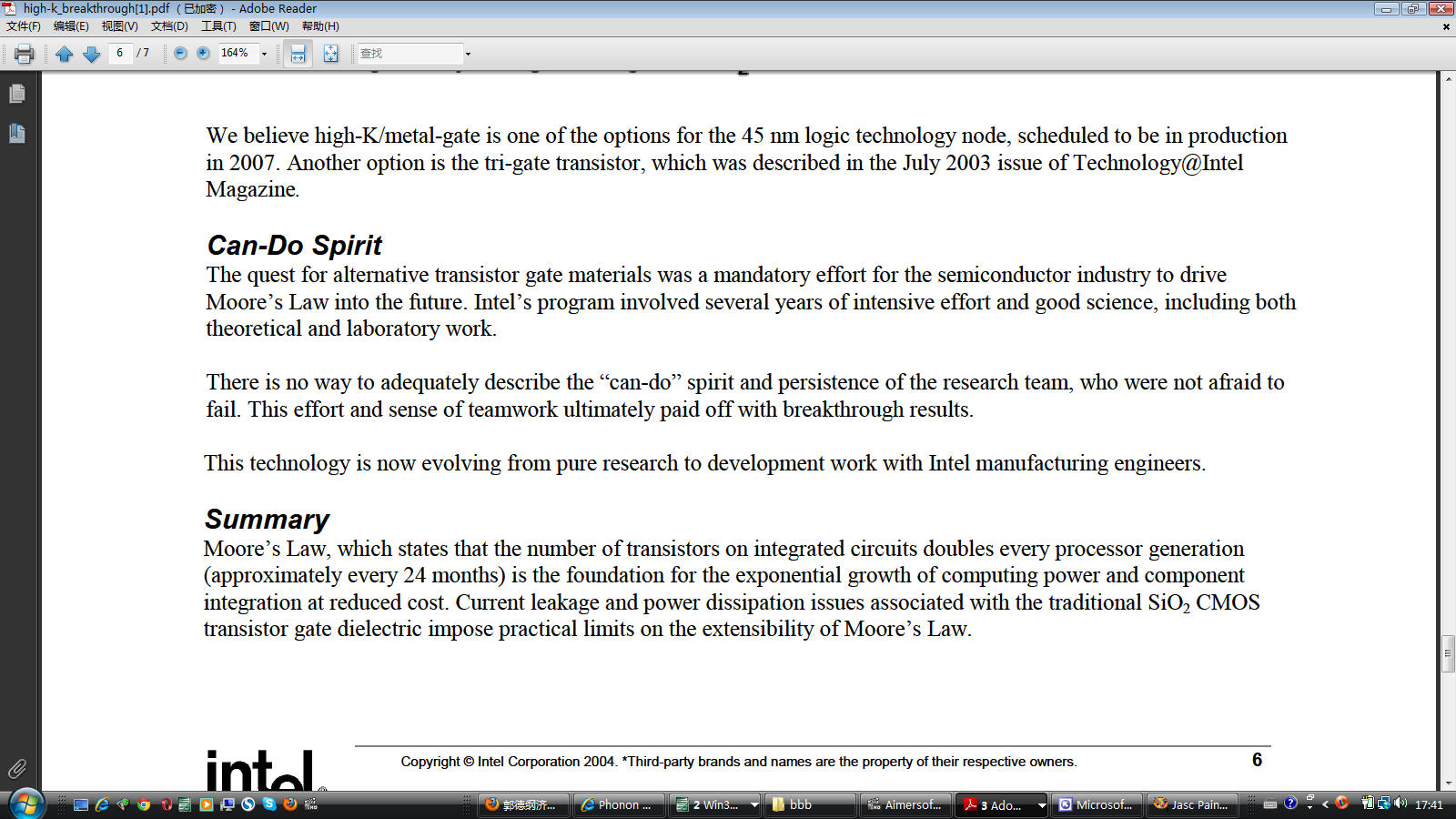This image showcases a computer screen with a sky-blue top bar that remains unreadable. The screen's left side features a black bar displaying two icons, possibly related to WordPress or document management, and a paperclip icon at the bottom. To the right of the black bar, there's a gray toolbar that includes an array of icons: a recognizable Adobe PDF icon, copy and print icons, two blue arrows facing upwards and downwards, and a box containing the number six. Below this toolbar is a section where font size can be adjusted.

In the main white section of the screen, there is a block of text discussing advanced semiconductor technology. The text reads as follows:

"We believe Hi-K Metal Gate is one of the options for the 45nm logic technology node scheduled to be in production in 2007. Another option is the Tri-Gate transistor, which was described in the July 2003 issue of Technology at Intel magazine. Can-do spirit. The quest for alternative transistor gate materials was a mandatory effort for the semiconductor industry to drive Moore's Law into the future. Intel's program involved several years of intensive effort and good science, including both theoretical and laboratory work. There is no way to adequately describe the 'can-do' spirit and persistence of the research team who were not afraid to fail. This effort and sense of teamwork ultimately paid off with breakthrough results. This technology is now evolving from pure research to development work with Intel manufacturing engineers. Summary: Moore's Law, which states that the number of transistors or integrated circuits doubles every generation approximately every 24 months, is the foundation for the exponential growth of computing power and component integration at reduced cost. Current leakage and power dissipation issues associated with the traditional SiO2 CMOS transistor gate dielectric impose practical limits on the extensibility of Moore's Law."

At the very bottom of the screen, there's an Intel copyright notice.